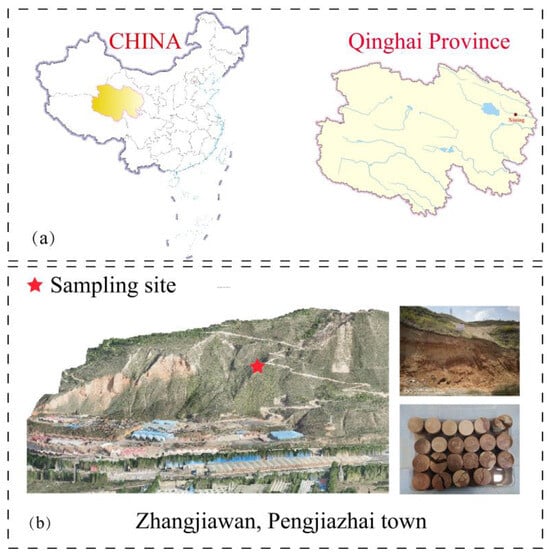The image is divided into two distinct halves. The top half features two maps: the map of China on the left labeled "CHINA" in capitalized red letters, and a more detailed map of Qinghai Province on the right, also labeled in red. These maps are separated by a dotted line and highlight Qinghai Province with a yellow section in the China map on the left. The bottom half, labeled by letter "B," presents three photographs. The large photograph on the left displays a site that appears to be a lumberyard, characterized by grassy and dirt areas with stacks of cut logs, and suggests significant forest clearing. Adjacent to this, on the right, are two smaller photographs, one depicting an area formerly populated with trees and now barren, and the other showing stacks of logs in detail. Below these images, there's a caption in black letters reading "Shengzhuangpingjiacai Town." The overall image is clear, with vibrant colors including yellow, light blue, green, brown, and red, and suggests a combination of digital creation and real photographs.